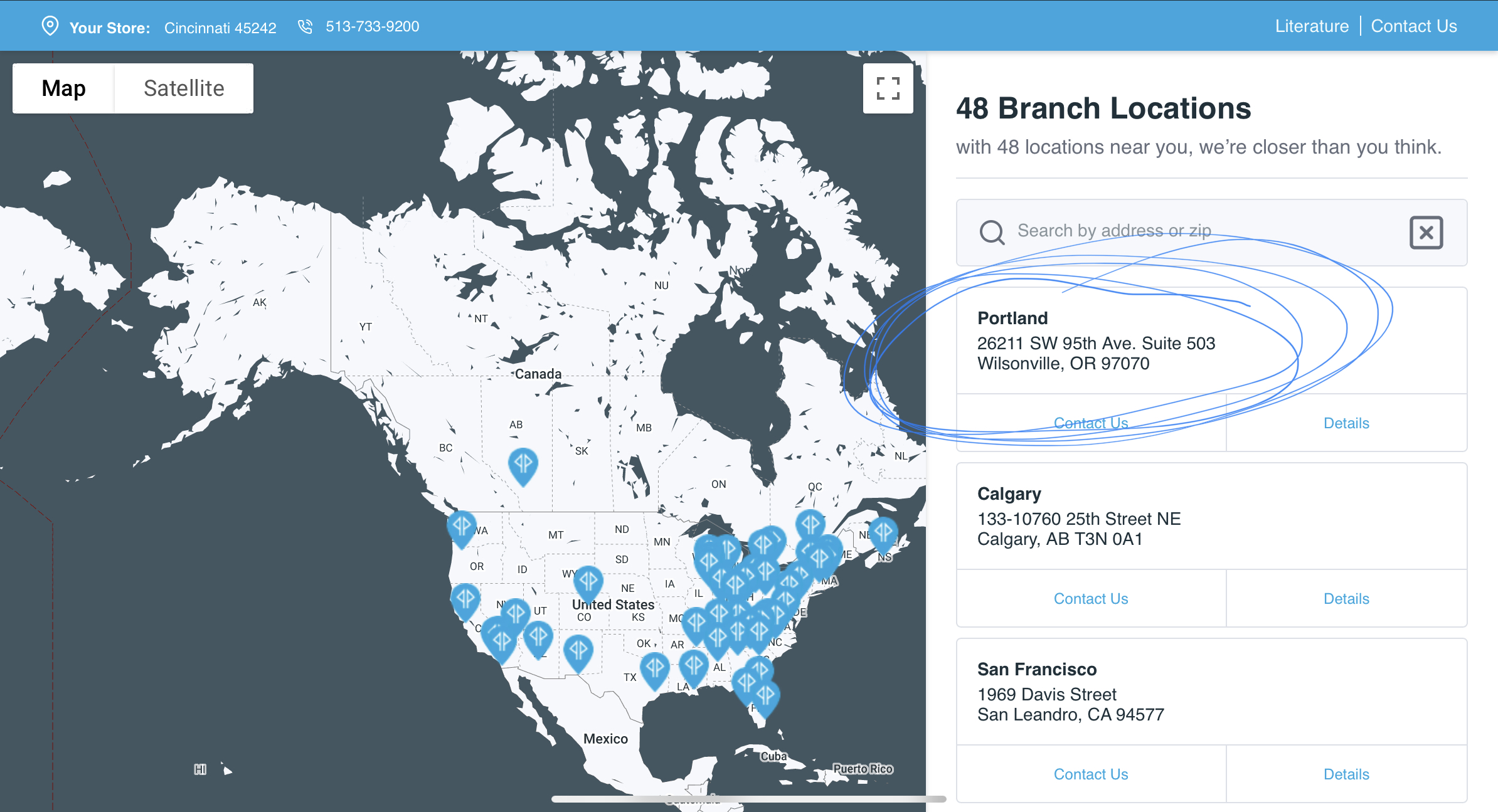In this image, you see a screenshot from a website. In the upper left-hand corner, it reads "Your Store Cincinnati 45242" along with the phone number "513-733-9200." In the upper right-hand corner, there are options labeled "Literature" and "Contact Us." On the left side of the image, there's a map displaying Canada, the United States, and a portion of Mexico. The map is dotted with numerous tiny blue map points, primarily clustered along the East Coast, with sparse points in California and Washington, and a single point in Canada. To the right of the map, text indicates "48 Branch Locations" followed by "With 48 locations near you or closer than you think." Below this message is a search bar where users can input their address or zip code. Three specific locations are highlighted: the first in Portland, the second in Calgary, and the third in San Francisco, California. Additionally, multiple circles have been drawn onto the screenshot, emphasizing certain areas.